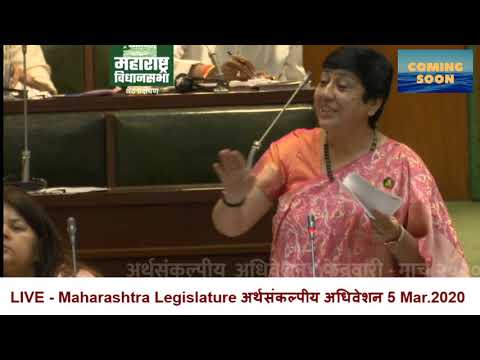In the center of this rectangular image, which measures approximately 3 inches wide and 2 inches tall, we observe a scene that appears to be taking place indoors, likely within a courtroom or interview setting during a political meeting in India. The image is bordered by black bands at the top and bottom and features a thin black vertical line along the left side. Just below the black footer, a white banner with red text reads, "Live Maharashtra Legislature" followed by some Indian script and the date "5 March 2020."

In the upper right-hand corner, there's a blue rectangle with yellow text stating "Coming Soon." The main subject of the photograph is a woman with short black hair and light brown skin, dressed in a traditional pink floral sari that also features orange and pink elements on the sleeves. She is viewed from about the waist up, positioned towards the left of the image, holding a sheet of paper in her left hand and gesturing with her right hand, palm facing upwards. Her facial expression suggests she is not amused.

In the background, several people are seated at desks or benches, with some writing on paper, indicating ongoing legislative or parliamentary activity. Additionally, part of another woman's head is visible in the lower left corner, positioned close to a microphone. The image includes a variety of colors, such as different shades of blue, white, pink, orange, tan, black, green, and brown. The overall composition captures a snapshot of live proceedings within the Maharashtra Legislature on the specified date.